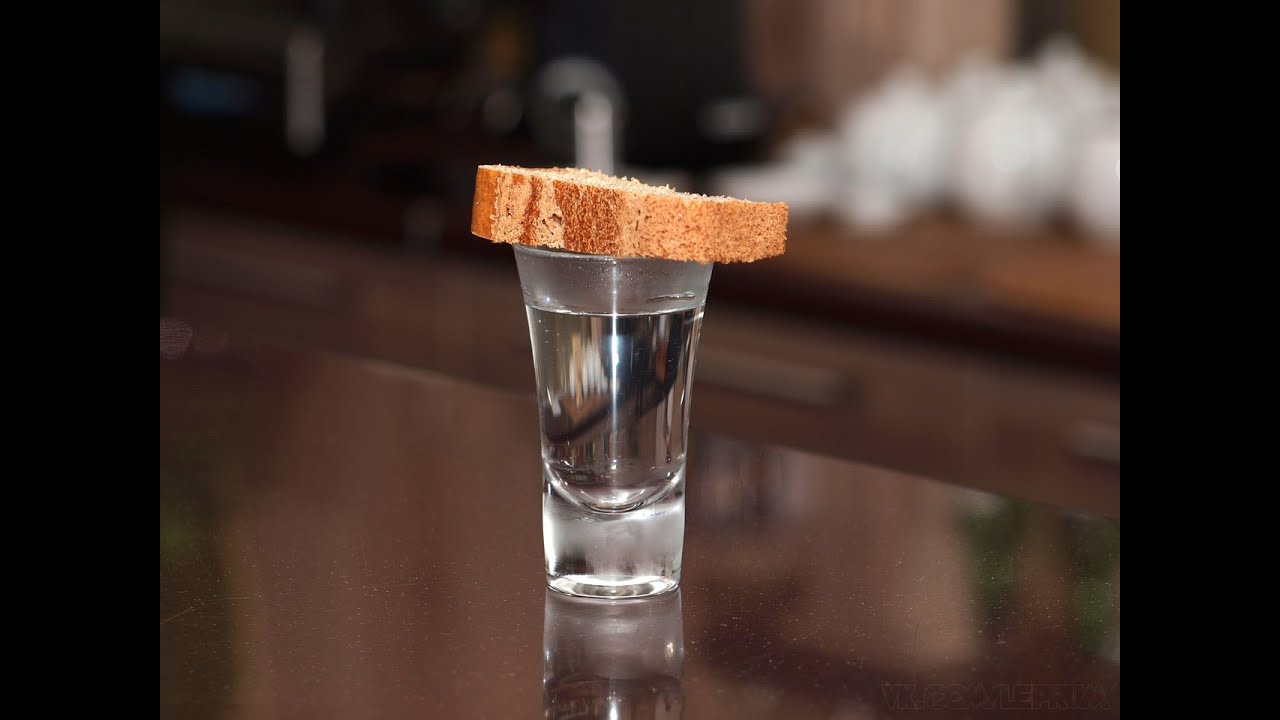The image depicts a clear shot glass filled with a clear liquid that rises approximately half an inch above the rim. A piece of bread with a brown crust and a lighter center is balanced on top of the shot glass. The glass and bread are positioned centrally on a dark, reflective kitchen countertop. In the blurred background, part of a cabinet and a countertop are visible, with some white mugs or cups discernible in the upper right corner. The setting features a kitchen with a brownish color theme.